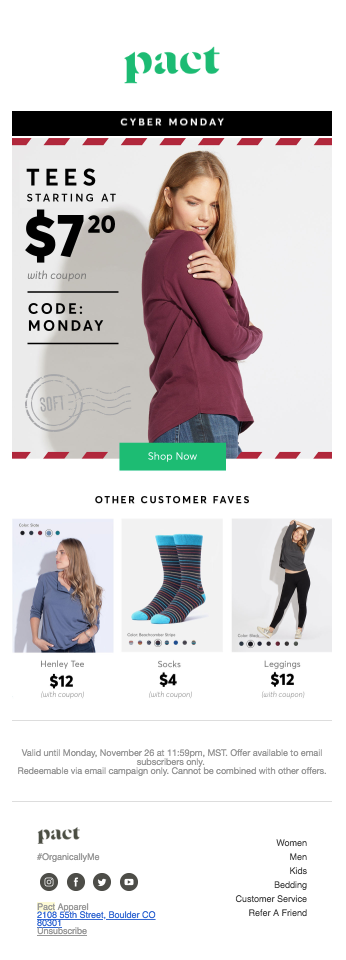At the top of the image, the word "PACT" is displayed in lowercase green letters, followed by the phrase "Cyber Monday." The image prominently features a woman with brown hair, wearing a long-sleeved burgundy shirt. Her hand rests gently near her shoulder, drawing attention to the soft fabric. Beside her, in bold uppercase black text, it reads "T's starting at $7.20 with coupon code MONDAY."

Below this, there is a green rectangle with the text "SHOP NOW," inviting viewers to take action. Adjacent to this, another image showcases a woman wearing a blue Henley T-shirt, her long brown hair cascading down. Beneath her, the Henley T-shirt is priced at $12.00. 

To the right, a pair of black striped socks with blue accents at the top and toes is displayed, priced at $4.00. Continuing downward, another image features a woman wearing black leggings and a dark gray shirt, with the leggings listed for $12.00.

The fine print notes the promotion's validity: "Valid until Monday, November 20th, at 11:59 PM. Redeemable via email campaign only; cannot be combined with other offers." At the bottom, the word "PACT" is again displayed, along with the hashtag "#originallyme."